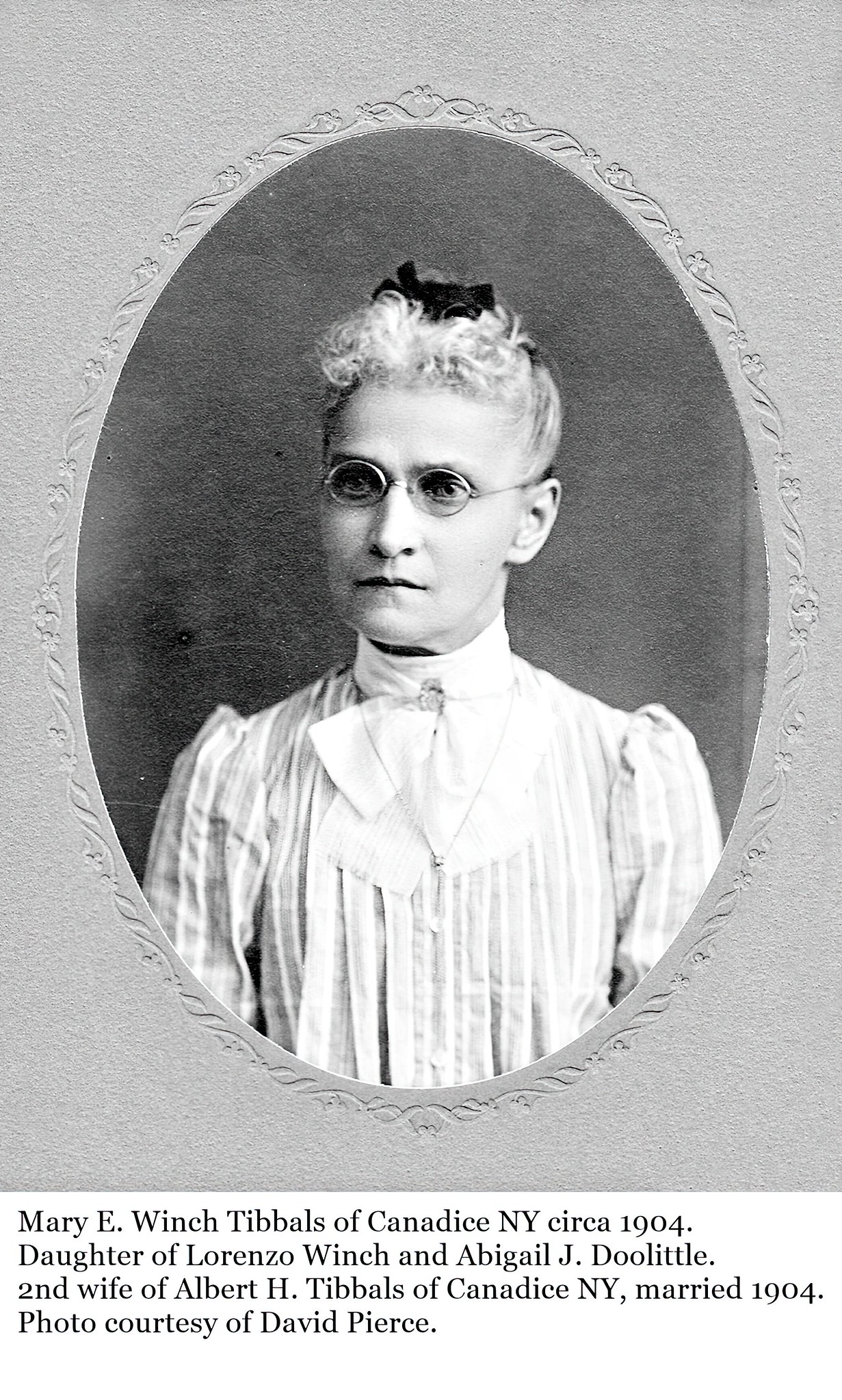This detailed black and white photograph, likely taken around 1904, depicts Mary E. Winch, the second wife of Albert H. Tibbles from Candice, New York. The portrait, courtesy of David Pierce, shows Mary dressed in a white lacy blouse adorned with a necklace and a brooch, pinning a ribbon at her neck. Sporting glasses and an attentive gaze into the camera, she is centrally positioned in the frame. The identification at the bottom of the image reads, "Mary E. Winch Tibbles of Candice, New York, circa 1904. Daughter of Lorenzo Winch and Abigail J. Doolittle." The photograph is a historical piece, hinting at Mary’s life and heritage, with the original frame featuring gray borders and black textual information.